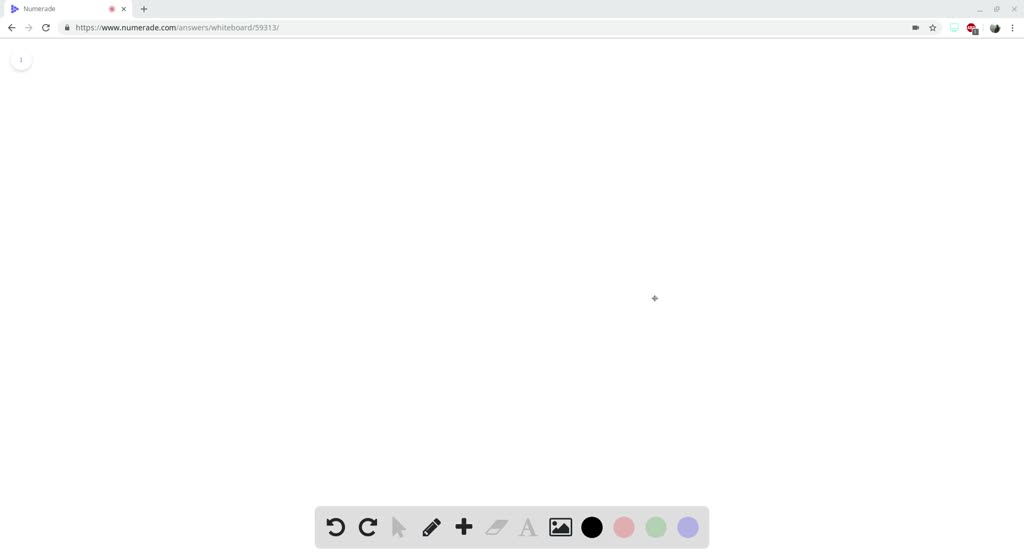This image, sourced from the website https://www.numeraid.com/, showcases a user interface (UI) filled with various navigational and functional elements. At the top, there are left and right arrow buttons, followed by a refresh button. A tab labeled "NumerAid" features a sleek design with a sideways triangle comprised of six blue dots. To the right of this tab, there is an "X" button for closing the page.

Further down towards the bottom of the interface, there are additional buttons for refreshing, indicated by directional arrows pointing left and right. A grey up arrow is prominently displayed, alongside a black pencil icon that likely represents an edit function. Additional buttons include an orange plus sign, a red plus sign, and a blue minus sign, each presumably serving different purposes within the interface. This detailed arrangement suggests a robust and user-friendly navigation system for the NumerAid platform.